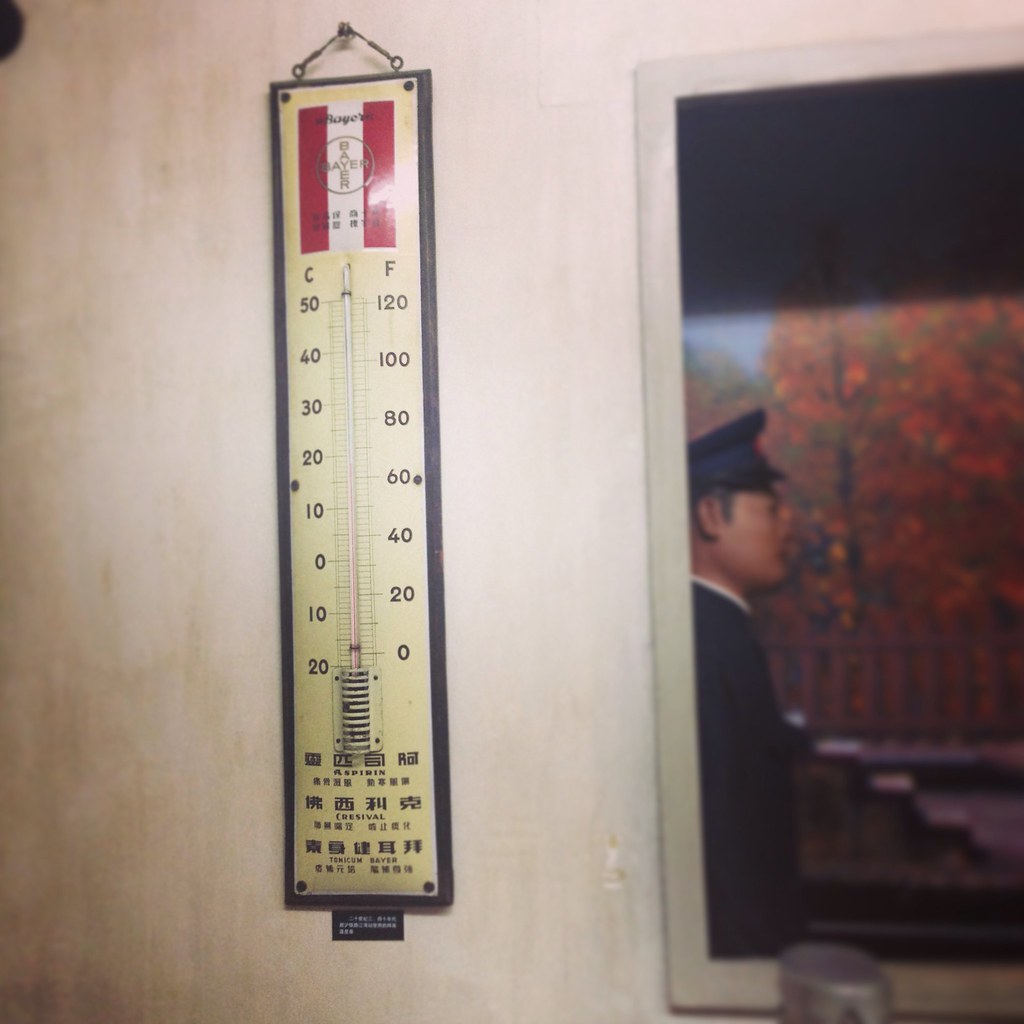In the image, we first notice a long rectangular sign hanging from a small nail. At the top of the sign, there is a depiction resembling a flag, featuring red and white stripes with a cross in the center. Below this image, there is a thermometer display with distinct temperature markings. The left side, denoted by the letter 'C' for Celsius, and the right side, marked by 'F' for Fahrenheit. The Celsius scale ranges downwards with numbers 50, 40, 30, 20, 10, 0, -10, and -20, while the Fahrenheit scale is listed as 120, 100, 80, 60, 40, 20, and 0. The thermometer is detailed with numerous black lines that indicate temperature increments.

Beneath the thermometer, there appears to be Chinese calligraphy, adding an element of cultural significance to the display. On the right side of the image, there is a painting encased in a white frame. The painting portrays a man in profile, donning a black military-style hat and a long-sleeved black coat. The background of the painting is an autumn scene with vibrant orange foliage and a set of visible steps leading into the scenery. The top portion of the painting is covered by a long black rectangular strip, and in the bottom right corner of the overall image, a silver lid can be observed.